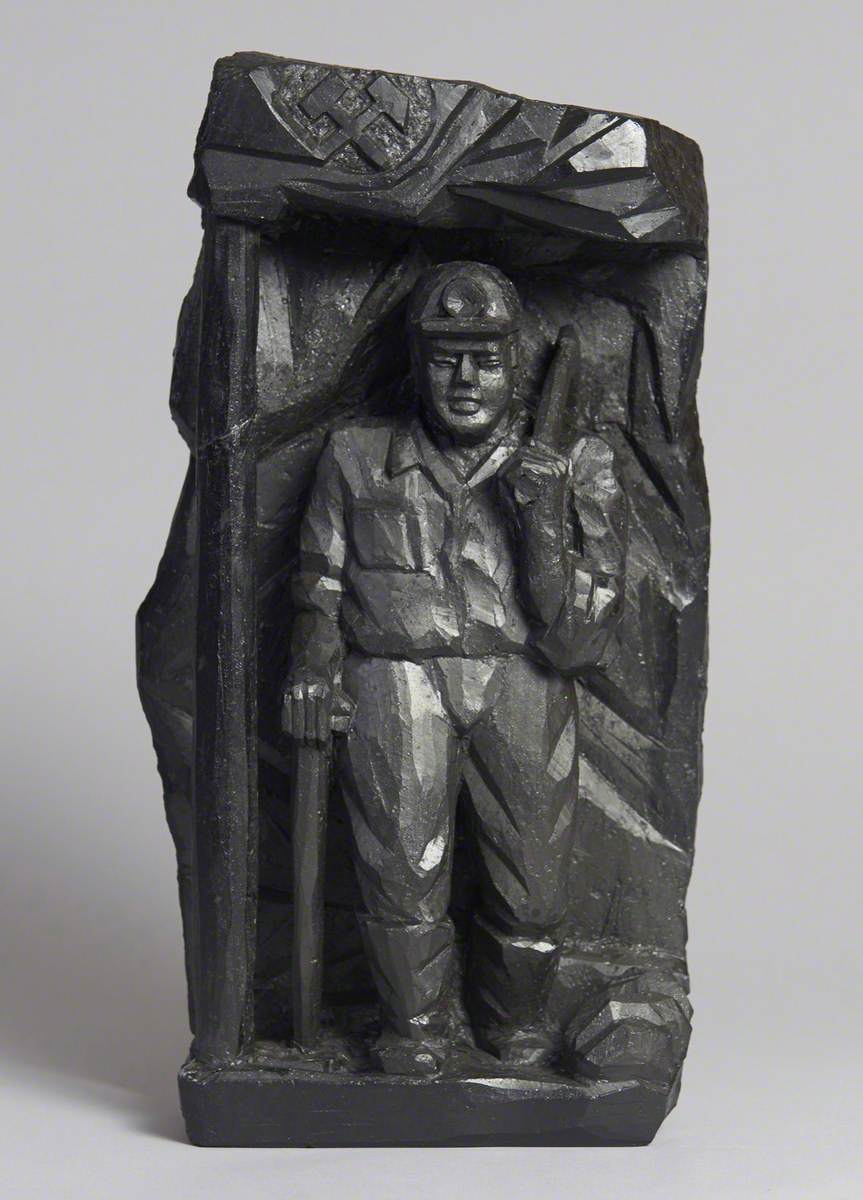This relief carving appears to be made from a dark, coal-colored stone, possibly blackstone or ebony, and stands against a grayish-charcoal background. The rectangular sculpture, approximately three feet high and two feet wide, depicts a coal miner in intricate detail. The miner, wearing a hard hat with a small torch or light affixed to the front, is dressed in a collared, tucked-in shirt, slacks, and boots. He leans on a pickaxe with his left hand, while his right hand rests on another tool. To his right, wooden posts support the ceiling of the depicted mine, adding to the scene's depth. Above him, two hammers are etched into the stone in a crisscross pattern, and a symbol is carved into the ceiling, enhancing the mining-themed tableau. The sculpture's glossy finish and meticulous details blend seamlessly into the matching background, creating a cohesive and lifelike representation of a coal miner's environment.